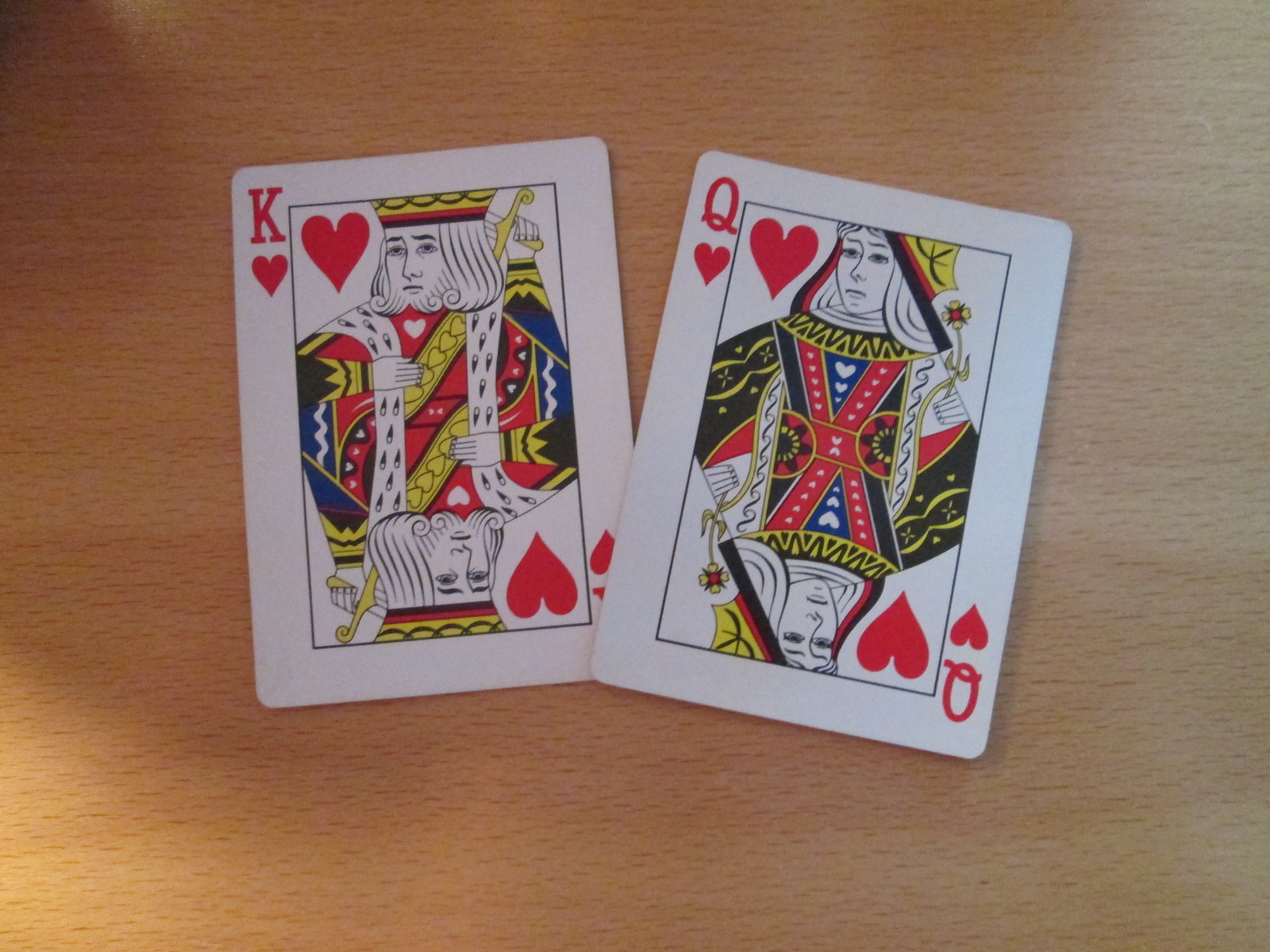A richly textured backdrop in shades of burnt orange, yellow, and tan captures the eye, resembling variances of light and shadow playing on a wooden surface. Positioned diagonally at a slight leftward tilt is the King of Hearts card. Directly to its right, overlapping the bottom right edge of the King, is the Queen of Hearts card, also set at a diagonal but tilted slightly to the right. Both playing cards feature traditional designs with white backgrounds. The King of Hearts is ornately dressed in red royal attire, with his regal face mirrored, gazing left from the top and right from the bottom of the image. The Queen of Hearts dons intricate red and blue clothing adorned with yellow ornamentation, her mirrored face looking to the left on the top side and to the right on the bottom. This carefully arranged pair of playing cards adds a layer of narrative richness to the already visually engaging scene.